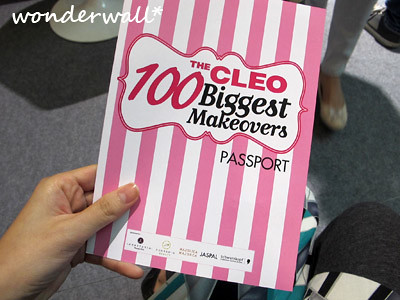In the photograph, a left hand prominently holds a card or book that features a pink and white striped cover. The central text on the cover, bordered in pink, reads "The 100 Clio Biggest Makeovers Passport." The words "The" and "Clio 100" are in pink, while "Biggest Makeovers" and "Passport" are in black. In the upper left corner of the cover, the scripted text "Wonder Wall" is visible, accompanied by a small asterisk.

The scene takes place outdoors on a gray ground illuminated by bright sunlight, which casts the shadows of the people present. In the image, only the lower legs of another person, wearing ballet slippers, are visible. Additionally, a blue bag, possibly a backpack, is seen on the ground. The composition suggests a casual setting, captured with thoughtful detail.